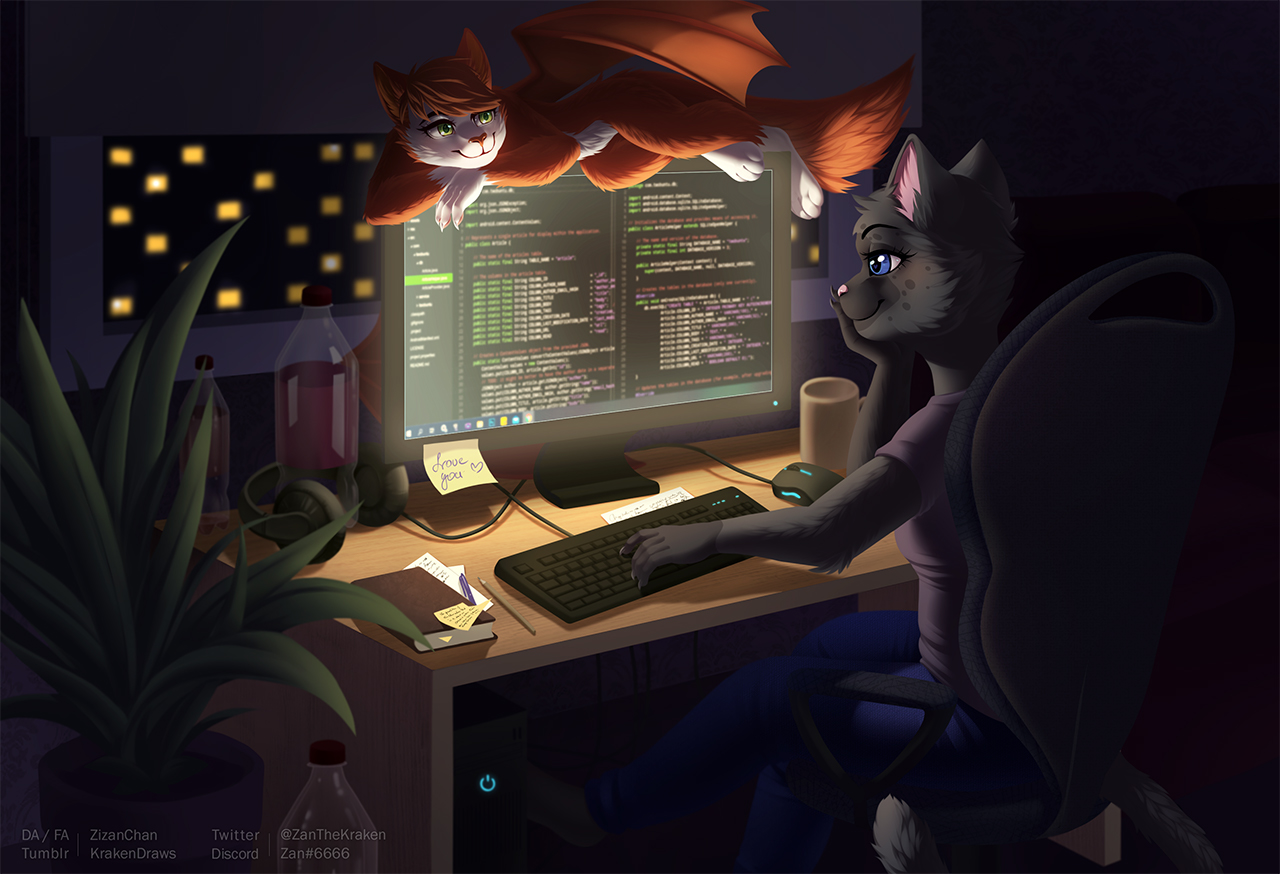In a vibrant cartoon image, two anthropomorphized cats are depicted in an office setting at night. The main focus is on a black cat, seated in a black computer chair at a brown desk, engrossed in typing on a black keyboard. The black cat, adorned in a short-sleeved purple t-shirt and blue pants, is thoughtfully resting its head on its right hand while its left hand actively taps away. Above the computer monitor, there's a smaller orange cat with distinctive orange bat wings, white face, paws, and belly, and green eyes peeking down, smiling at the typing cat. The orange cat has a playful tuft of orange hair cascading over its face. On the left side of the image, a green plant adds a touch of nature, while behind the scene, a large window reveals city lights cutting through the night sky. A soda bottle sits on the desk, and a yellow post-it note on the monitor sweetly reads "love you" adorned with a small heart. The screen also bears the digital signature, “D-A-F-A Cezanne Chan, Tumblr and Kraken Draws, Twitter at ZanTheKraken, Discord at Zan, hashtag 6666,” in light print at the lower left-hand corner.